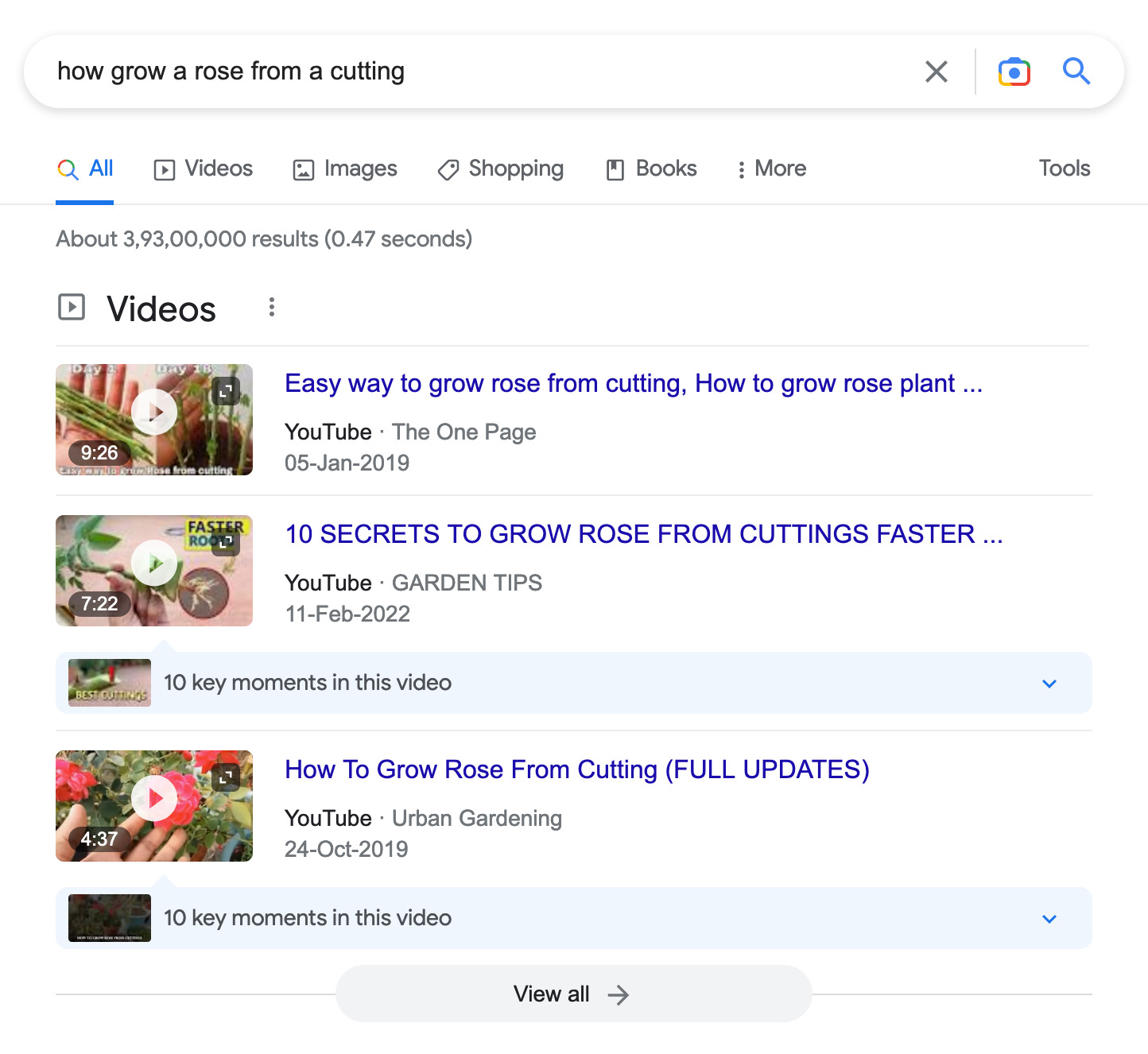This image is a detailed screenshot of a Google search results page viewed on a smartphone. At the top, the search query "how to grow a rose from a cutting" is prominently displayed in a gray font within the search box. Directly below the search box, a navigation bar features various categories including "All," "Videos," "Images," "Shopping," "Books," a set of three vertical dots indicating more options, and "Tools." The "All" category is highlighted in blue, showing that it has been selected.

To the far left of this navigation bar, the total number of search results is displayed: about 3,093,930,000 results in 0.47 seconds. Below this information, the page is divided into sections starting with "Videos."

Three video thumbnails are prominently featured under the "Videos" section. The titles of these videos are:
1. "Easy Way to Grow Rose from Cutting | How to Grow Rose Plant"
2. "10 Secrets to Grow Rose from Cuttings Faster"
3. "How to Grow Rose from Cutting (FULL UPDATES)"

Each video title suggests various methods and tips for growing roses from cuttings, with the third title emphasizing comprehensive details with "FULL UPDATES" in capital letters.